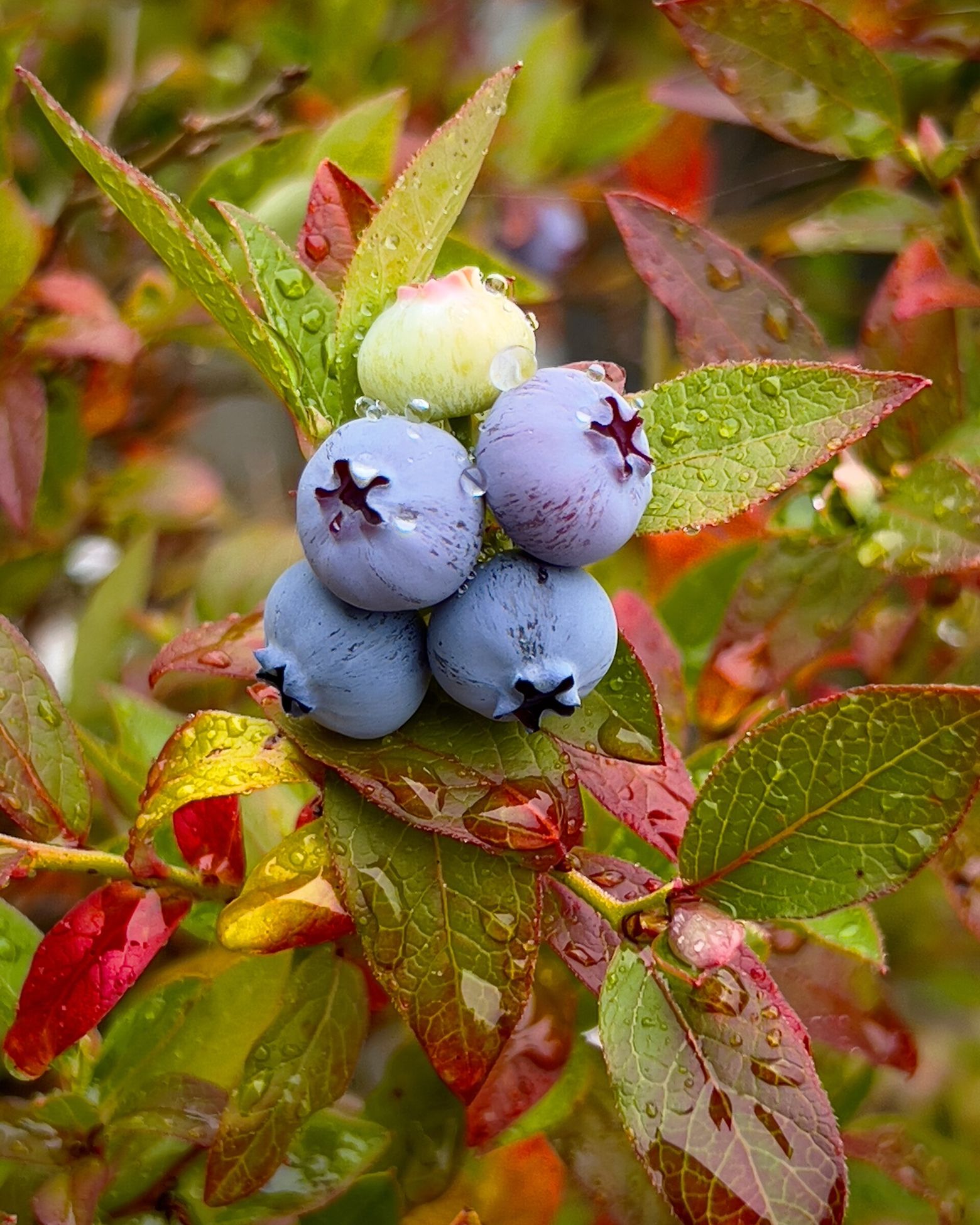This close-up image captures a cluster of wild berries growing on a vibrant plant. The plant features green leaves with red edges and a yellow stem. The berries are prominently displayed in the center, with four of them fully ripe and showcasing a light blue-lilac hue with maroon and white speckles. One berry on the top is still unripe, appearing green. The scene is set after a rain, with water droplets clinging to the leaves and berries, adding a fresh, dewy appearance. A delicate spider web is visible in the bottom right corner of the image, enhancing the natural feel of the setting. In the background, numerous other branches can be seen, giving context to this detailed snapshot of the plant.